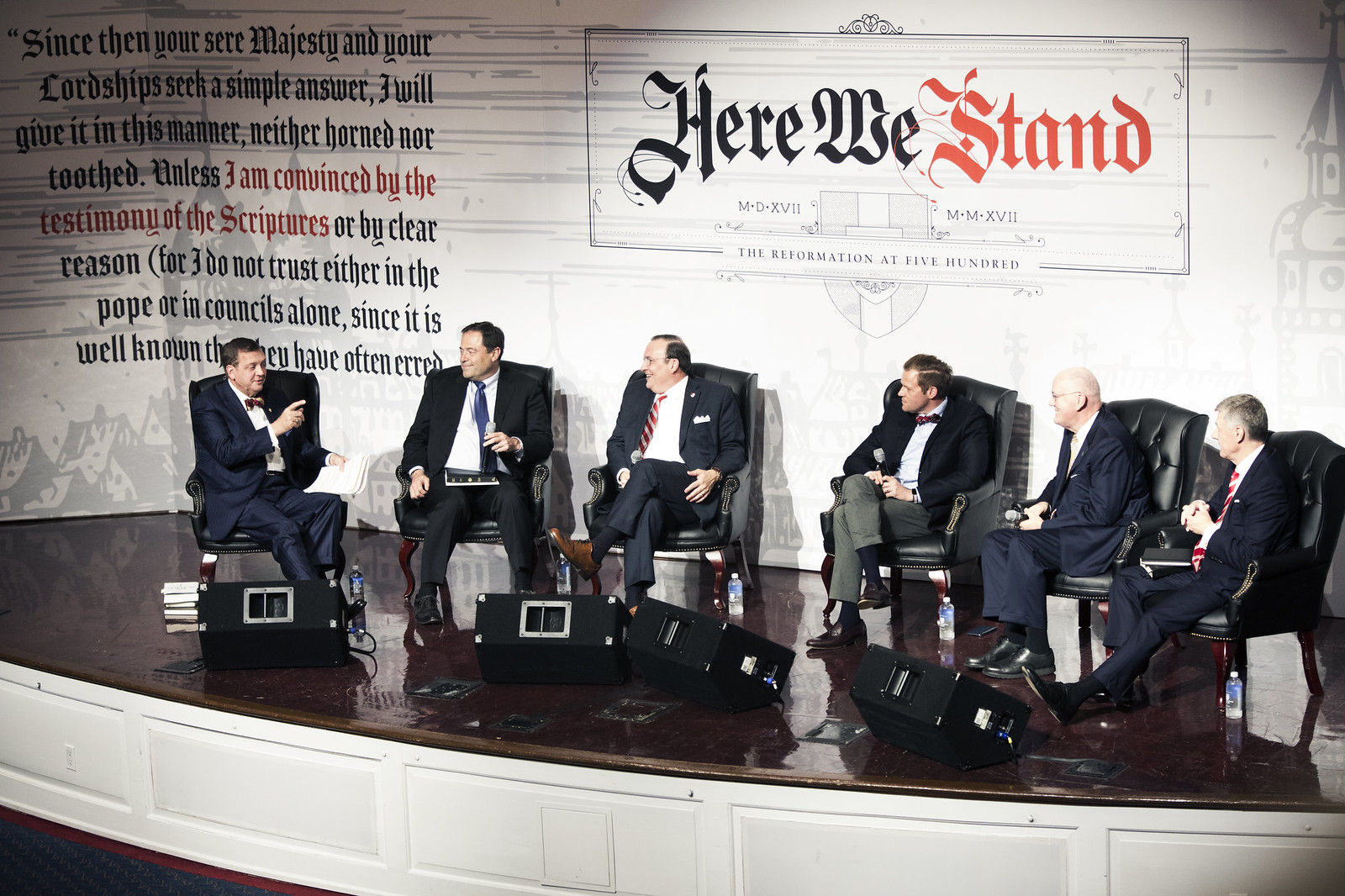The image depicts a photograph of six middle-aged white men sitting on a large, glossy wooden stage, seemingly engaged in a conference or a political discussion. All the men are dressed in dark suits, either black or navy blue, and are seated in high-end leather chairs with wooden legs. Most of them are wearing ties, with some donning navy blue or red ties, and a few opting for bow ties. The men are arranged with three on the left and three on the right, and one man on the far left is visibly mid-conversation, gesturing with one hand while holding a sheet of paper in the other. The other five men are facing him, appearing to listen and smile in agreement.

In the foreground, there are four black speakers positioned towards the men on stage. The backdrop features a cream-colored wall with prominently displayed text in black and red. To the left, a paragraph in black font, partially highlighted in red, reads: "Since then, your majesty and your lordships seek a simple answer, I will give it in this manner, neither horned nor toothed. Unless I am convinced by the testimony of the scriptures or by clear reason, for I do not trust either in pope or councils alone, since it is well known they have often erred." Above this writing, a black rectangle contains the text "Here We Stand" with "Here We" in black and "Stand" in light red, followed by the smaller black text, "The Reformation at 500," along with some Roman numerals. The photograph captures a moment of engaged dialogue against a backdrop suggestive of a historical or religious theme.